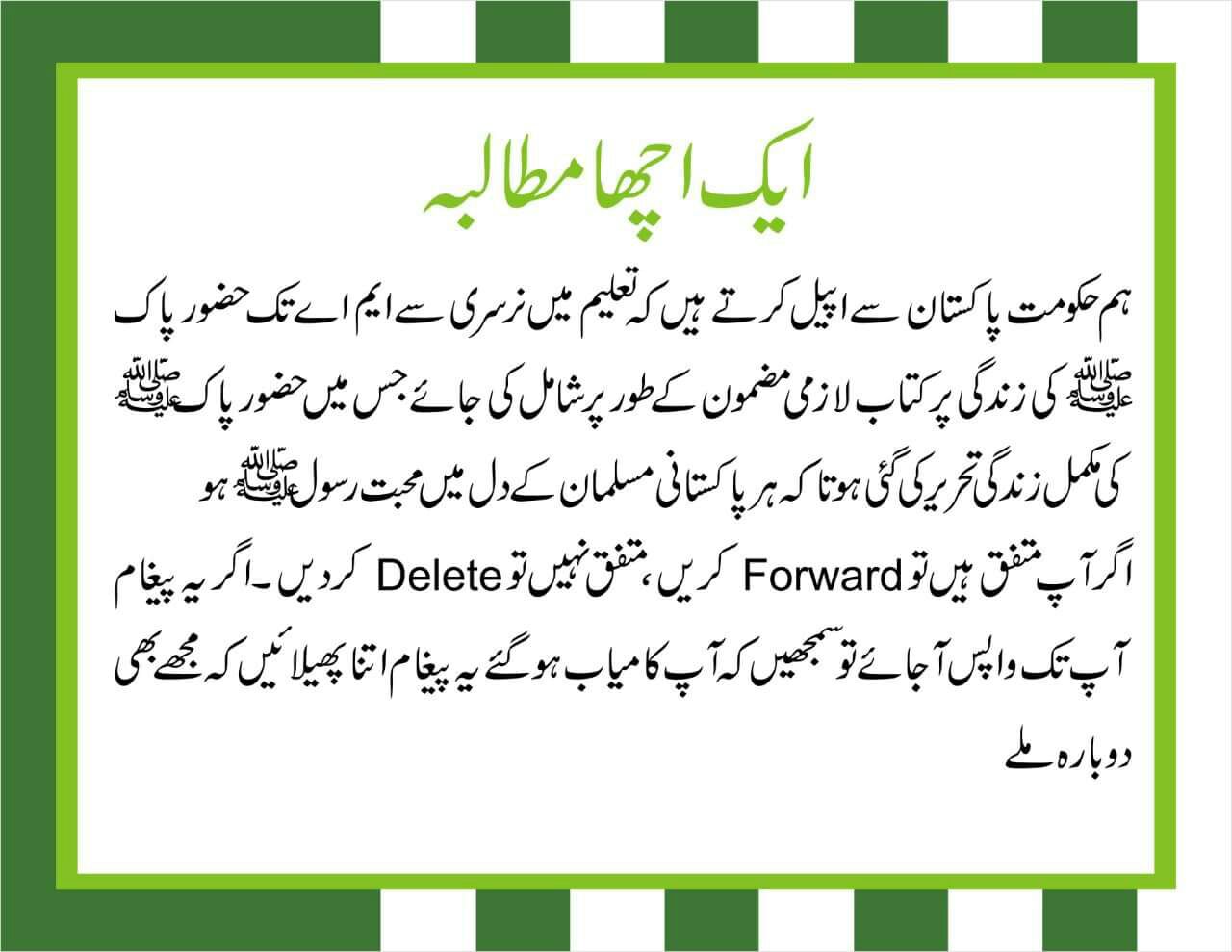The image depicts a rectangular graphic predominantly featuring Arabic script. The central part of the image is a white rectangle bordered by a green frame, inside which multiple rows of Arabic text are written. The second row from the bottom includes the only English words in the piece: "delete" on the left side and "forward" on the right. Behind the white rectangle, there is a pattern of green and white stripes, with the leftmost stripe being significantly thicker. At the top of the image, there is a green title, although it is hard to discern exactly what it says. The overall design includes varying shades of green, with both light and dark green elements creating a distinct border and striped background. The composition suggests it might be a card, poster, or some form of written document.